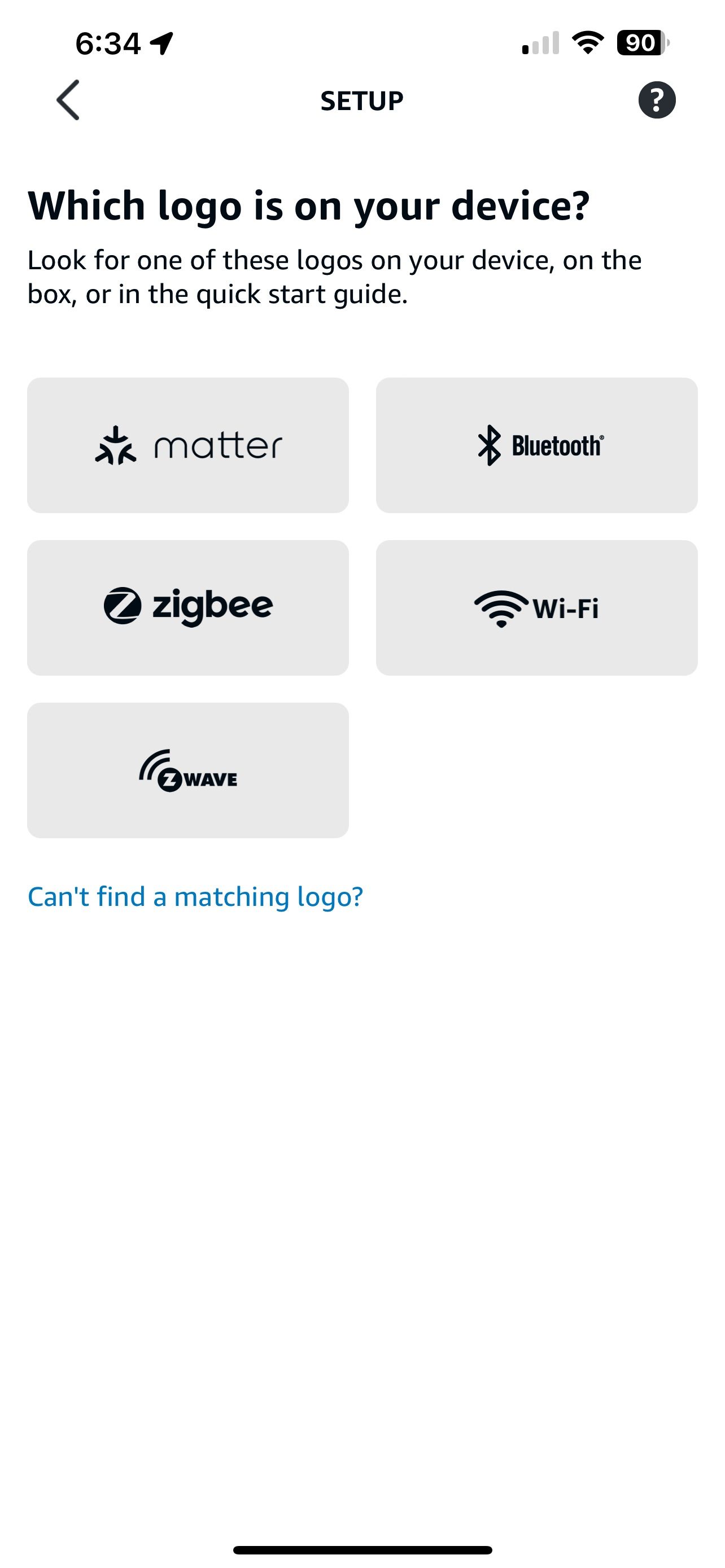A screen capture of a cell phone setup screen, likely from an international device, is displayed. The status bar at the top shows the date and time (6:34), along with icons indicating location services, Wi-Fi connectivity, cellular signal, and a battery level at 90%. Below this, the screen prompts the user with "Setup?" followed by "Which logo is on your device?". It advises the user to look for one of the following logos on their device, box, or quick start guide: Matter, Bluetooth, Zigbee, Wi-Fi, and Z-Wave. Additionally, there is a query at the bottom asking "Can't find a matching logo?" suggesting further steps to continue with the device setup. This screen capture visually guides the user through the initial setup process by identifying compatible connectivity standards.